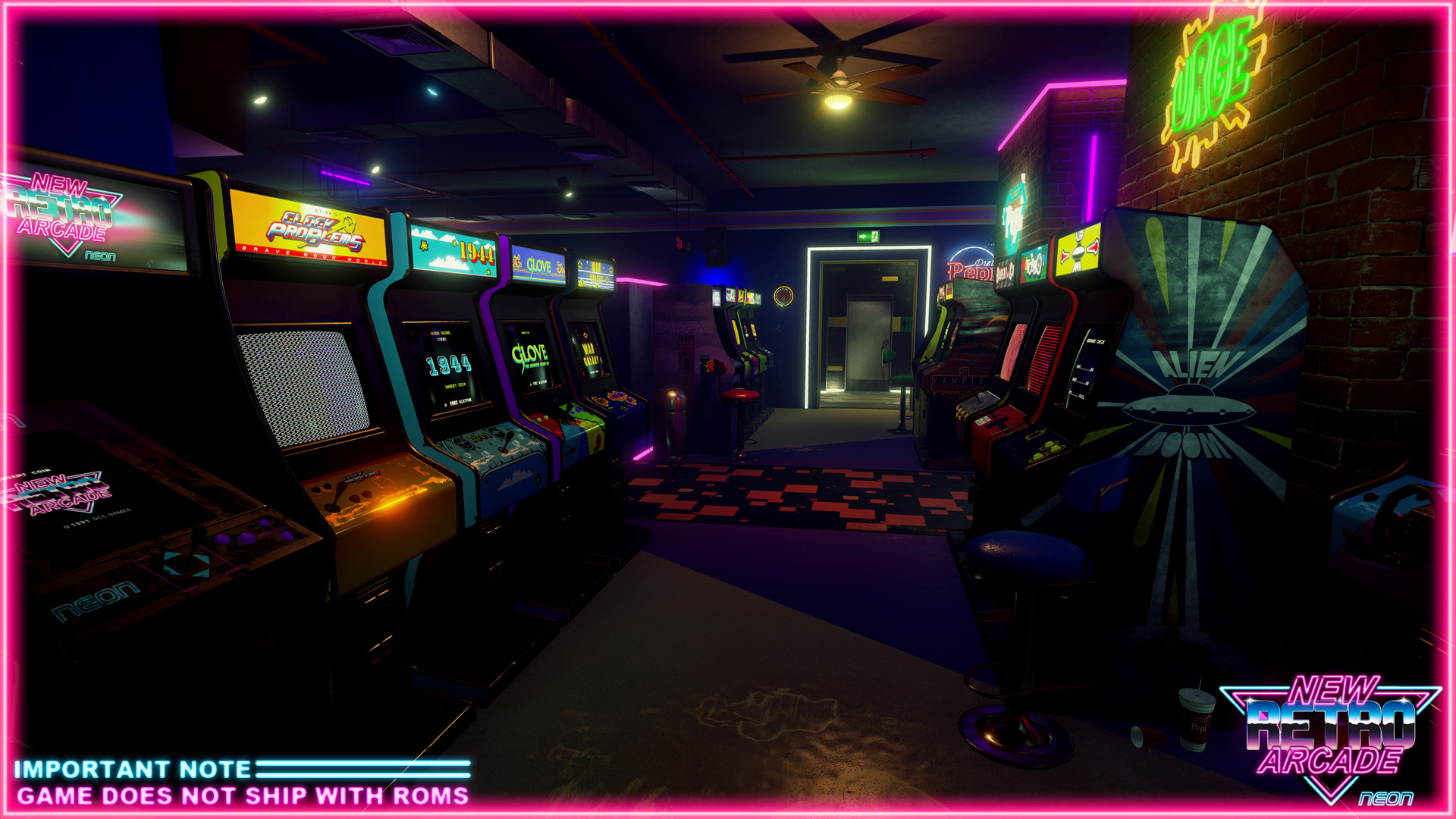The image is an intriguing, somewhat dimly lit scene inside an arcade depicted in a computer-generated format with a neon pink border accentuating its horizontal rectangular shape. The bottom right corner captions "New Retro Arcade, Neon," while the bottom left notes that the "game does not ship with ROMs," hinting that this might be part of a promotional material for a video game. The simulated arcade environment is incredibly realistic, featuring rows of classic stand-up arcade machines stretching into the distance on both sides, evoking the ambiance of an authentic 80s arcade. To the right, a red brick wall supports a series of neon signs and trim, including a prominent machine labeled "Alien." The left side mirrors this with more arcade games, highlighted by a black and red checkered rug running along the concrete-gray floor. The ceiling is peppered with subtle lighting to complement the neon glow, and a door can be glimpsed at the back center of the room, completing the retro-futuristic vibe.